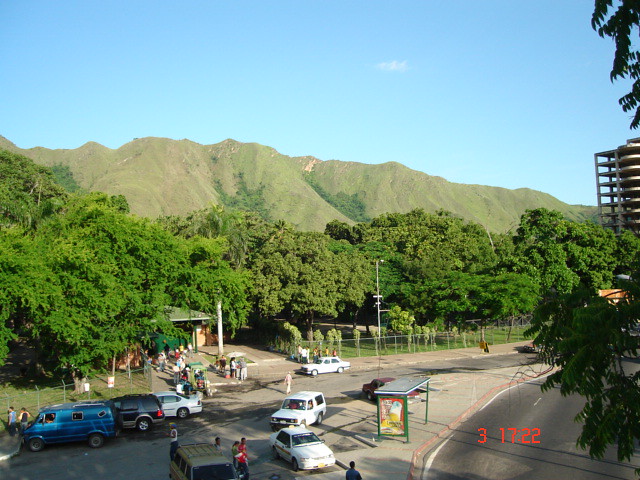This photograph captures an aerial view of a bustling park area, with a road that forks into two directions. The left fork curves closer to the viewer, while the right fork angles slightly diagonally. Along the right side of the road, a series of cars, including multiple white sedans, a white SUV, a blue van, and others, can be seen parked or in motion, seemingly searching for parking spots. A lively sidewalk is filled with people, some within the parking lot and others near a bus stop on the right. The shelter at the bus stop is green, and there’s a cluster of people around what appears to be a building, though obscured by the dense foliage.

The scene is defined by lush greenery, with large trees, bushes, and hedges throughout a grassy park area. In the background, rolling foothills covered in verdant trees give way to a brilliant blue sky. On the image, a red watermark is visible, displaying the numbers 3, 10, or possibly 17, 22. This park setting, enriched by both natural and urban elements, creates a harmonious and vivid depiction of daily life against a picturesque backdrop.